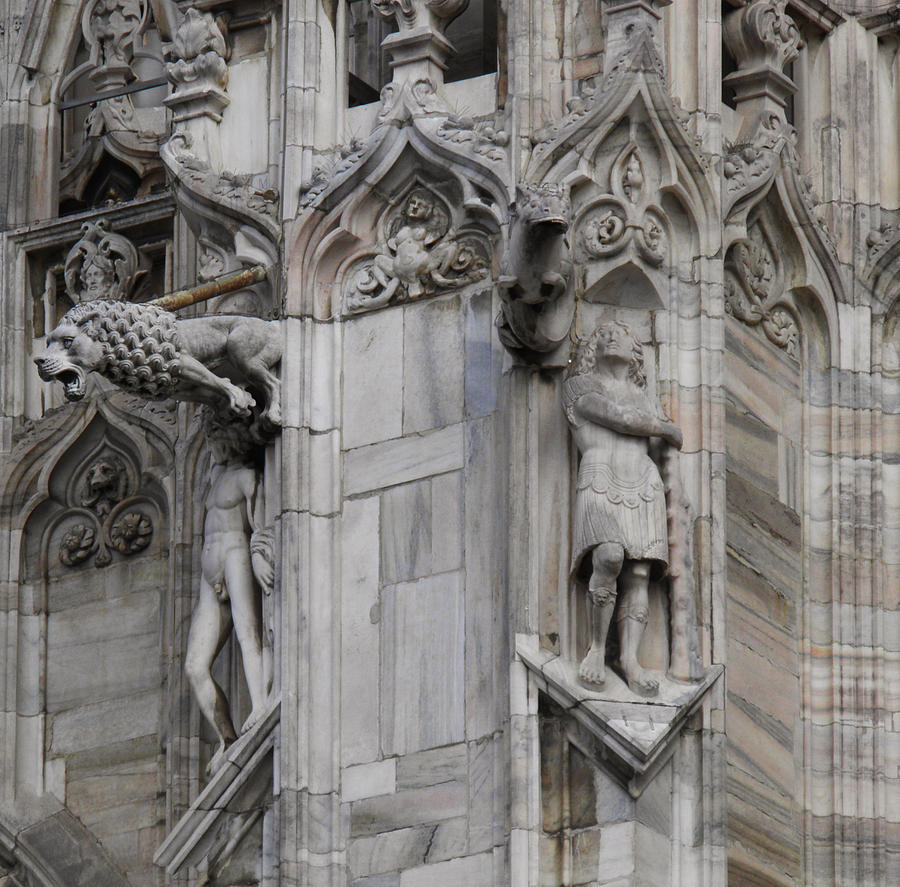This image showcases a meticulously carved section of an elegant, ornate European building, likely a church or a palace. The architecture features an array of intricate stone or marble artwork, blending hues of beige, blue-gray, and orange. Prominent among the carvings are two human statues: one on the left depicted fully nude and another on the right adorned in a Roman-themed outfit. Above the nude figure, a lion statue with its mouth wide open dramatically juts out from the facade. Higher up, a variety of smaller decorative elements and pointy archways add to the grandeur of the structure. This detailed close-up captures just a small portion of what is evidently a much larger, stunningly elaborate edifice.